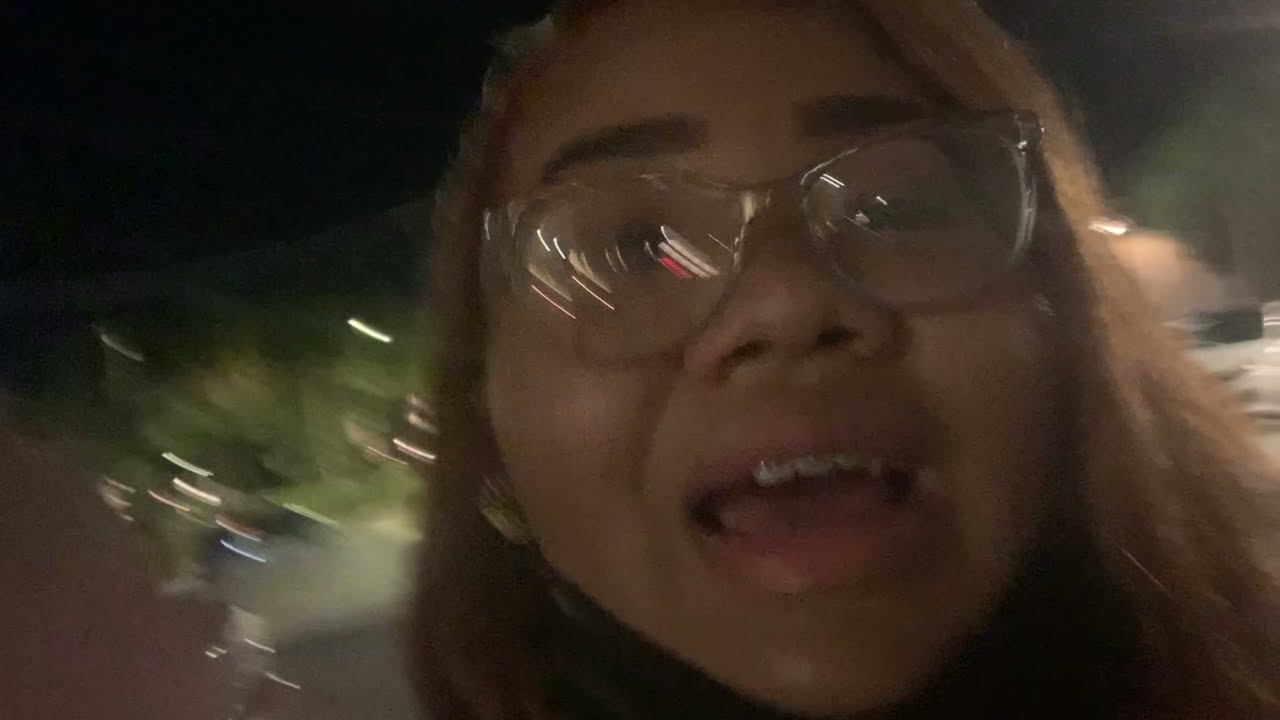The image is a very close-up selfie of a young African-American woman, possibly a teenager or young adult. The photograph is blurry, as if taken in motion, with most of the frame occupied by her face, starting at the forehead and ending just below the chin. She has large, pink lips, and her mouth is open, revealing upper teeth adorned with metal braces. Her thick eyebrows are short, and her nostrils are noticeably large. She appears to be wearing clear, 80s-style glasses that reflect bits of beige, red, and white light. Her long hair is dyed a chestnut brown with a hint of reddish color. The expression on her face suggests distress or surprise. The background is mostly indistinct due to the blur, but it seems like she is in a dark residential area with some lighting and possibly trees and bushes visible.